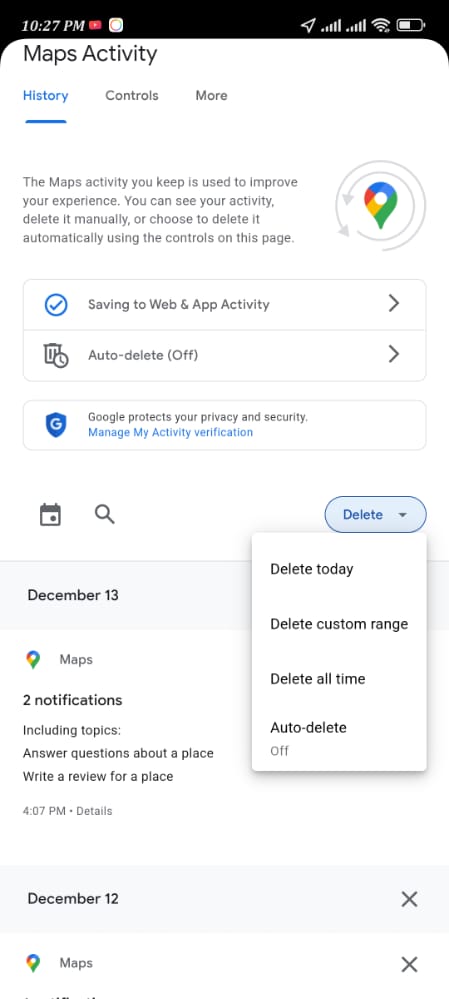This image is a cell phone screenshot with a clean white background. At the top, there is a black rectangle displaying various cell phone icons. Below this, in the upper left-hand corner, bold black text reads "Maps Activity."

A couple of lines down, there are three horizontally arranged menu items. The first menu item, "History," is highlighted in blue and underlined. The second menu item, "Controls," and the third, "More," are both in black.

Approximately four lines down, there is a paragraph written in gray text that states: "The Maps Activity you keep is used to improve your experience. You can see your activity, delete it manually, or choose to delete it automatically using the controls on this page." Adjacent to this paragraph is the Google Map pin icon, outlined by two incomplete gray circles with arrows on the left side.

Below the paragraph, there is a rectangle containing two lines, each with an icon on the left. The first line, in gray, reads "Saving to Web & App Activity," while the second line reads "Auto-delete (Off)." Both lines feature a right-pointing gray arrow resembling a sideways "V."

Further down, there is a white rectangle with a blue shield icon on the left. Next to it, text reads, "Google protects your privacy and security." Below this, in blue, it says, "Manage My Activity Verification." Adjacent to this, on the right, are calendar and magnifying glass icons. Finally, there is an oval-shaped delete button with a down arrow which has been pressed, revealing a white pop-up box. This pop-up box contains four lines of black text: "Delete Today," "Delete Custom Range," "Delete All Time," and "Auto-Delete."